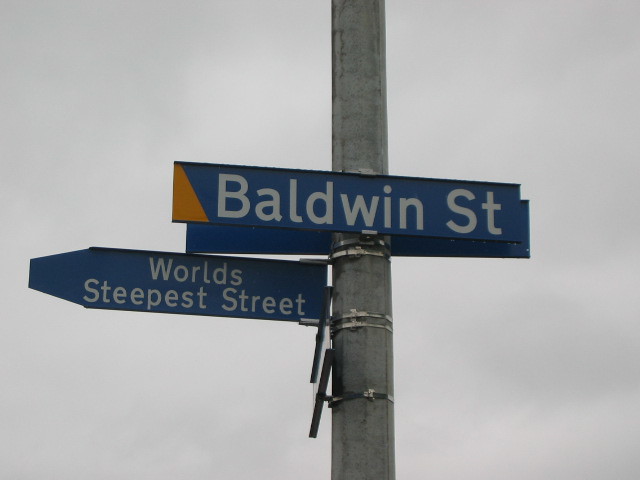The photograph captures a close-up of a tall silver metal street post on a cloud-covered, gray day. At the top of the post, there's a street sign adorned with a golden left border and blue background, prominently displaying "Baldwin St" in white letters. Just below, another sign in a blue, arrow-like shape reads "World's Steepest Street," also in white lettering. The pole has additional signs strapped to it with zinc brackets, but only their backs are visible, making them illegible. The overall scene is illuminated by the soft daylight, adding a stark contrast to the gray sky.